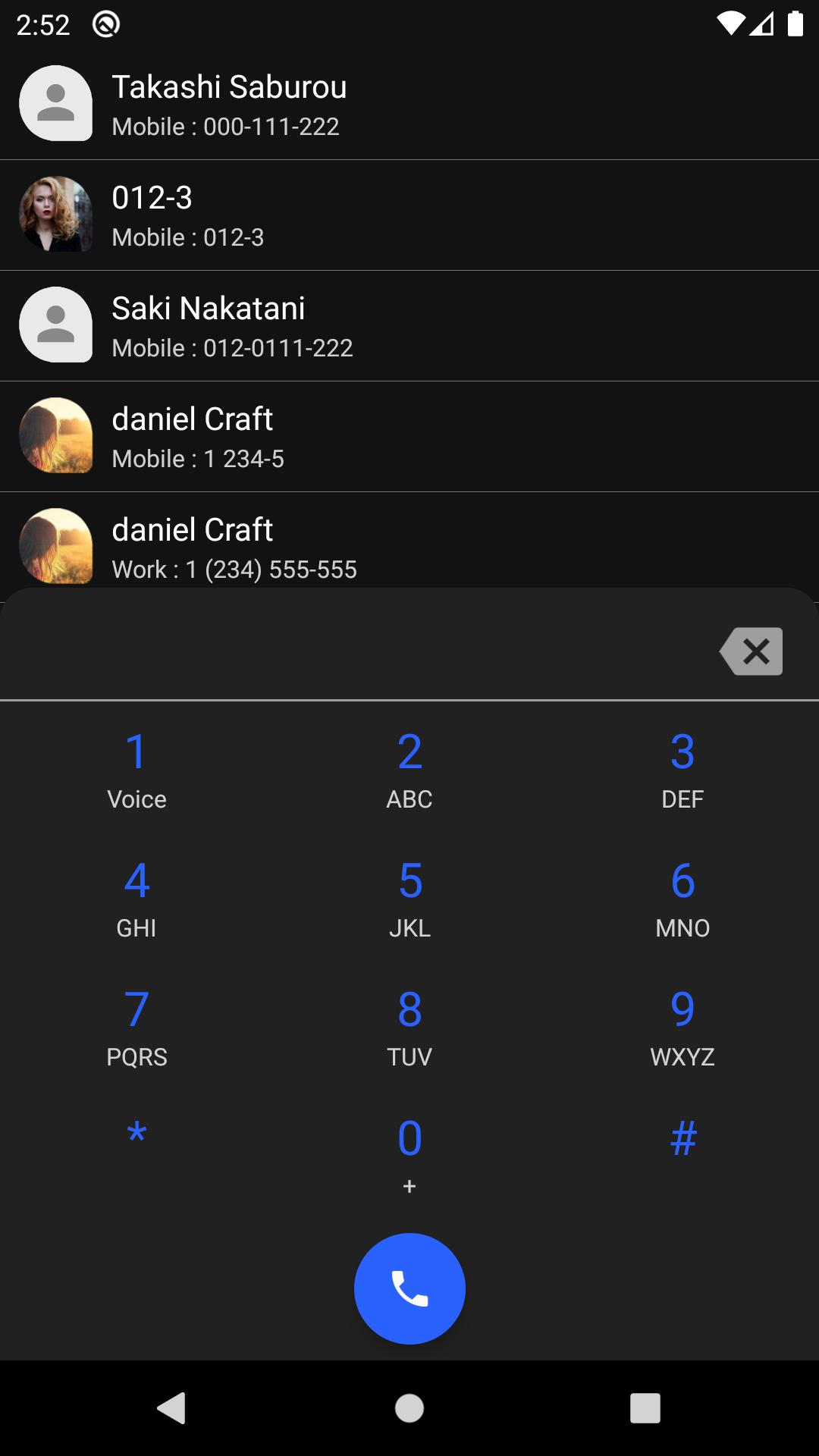The image displays a phone screen user interface organized into sections. At the top, the screen shows the name "Takashi Saburo" accompanied by a blank icon. Below this entry is a contact number, listed as "012-3".

On the left side of the screen, next in the contact list, is a photo of a girl with thick red hair, identified as Saki Nakatani. She is described as white. Saki Nakatani's name appears below her picture, but no additional icon is chosen for this contact.

Following Saki Nakatani is the contact "Daniel Craft," listed twice. The first entry for Daniel Craft includes an icon on the left, but the picture is unclear. The first entry likely corresponds to his mobile number, while the second entry lists his work number. Each of the four contacts—Takashi Saburo, Saki Nakatani, and both entries for Daniel Craft—has their mobile number displayed below their names.

At the bottom of the screen, the phone pad is displayed. The pad contains numbers 1 through 0, the pound sign (#), and the star sign (*), all written in blue text. Below each number, the letters of the alphabet are shown in white text. At the very bottom of the screen, there's a round, oval-shaped blue button featuring a white phone icon in the center, typically used to initiate a call.